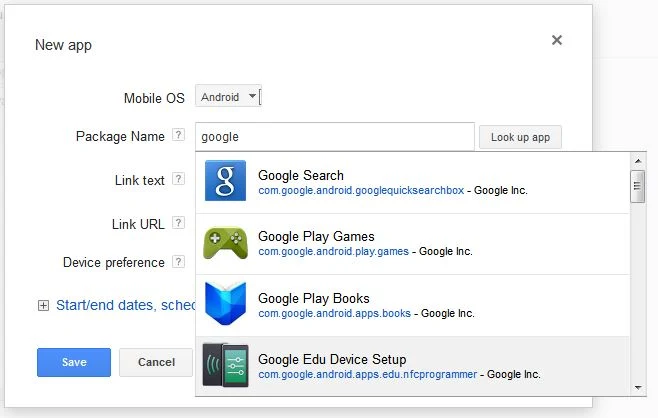The image displays a user interface of a new application named "Topless," compatible with Android devices. The package name for the application is 'google'. The interface prominently features a search functionality with a Google search bar, identified with the package `com.google.android.googlequicksearchbox`, linked to a Google URL. 

Beneath the search bar, the interface is organized into four rows showcasing various Google-related services: 

1. Google Search (`com.google.android.googlequicksearchbox`)
2. Google Play Games (`com.google.android.play.games`) 
3. Google Play Books (`com.google.android.apps.books`)
4. Google Edu Device Setup (`com.google.android.apps.edu.nfcprogrammer`)

Each service entry includes a corresponding Google link for quick access. 

The app includes features for device preferences and the ability to input start and end dates, likely for filtering or scheduling purposes. Visible on the interface is a "Cancel" button within a rectangular section. Additionally, a vertical scrollbar is present, gray in color along the edges, and contrasted against a white background, allowing for navigation through the content. The design and layout of the application contribute to a modern and efficient user experience.